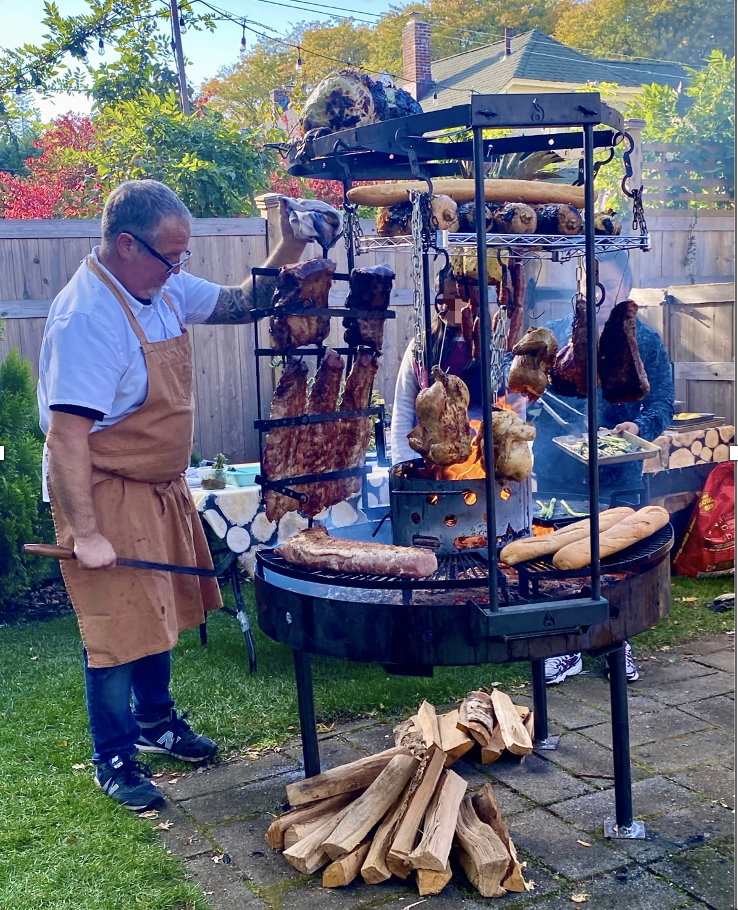This image captures a lively backyard scene shaped as a vertical rectangle, resembling a realistic photograph taken outdoors. In the background, a light blue sky occupies the top left, accentuated by a picturesque tree line adorned with green, red, and yellow leaves. A telephone line and the roof of a house subtly underscore the suburban setting. The foreground reveals a well-kept green lawn and a light wooden privacy fence that encloses the area, alongside a cement patio on the right side. 

Dominating the scene, there is a very large, vertical, black smoker or barbecue grill with a circular base and vertical shelves, laden with an array of meats—racks of ribs, possibly a chicken or turkey, and other cuts—hanging and cooking over an evident flame. 

The main figure in the scene is an adult man with white skin, dressed in blue jeans, a light blue short-sleeved shirt, a brown apron, and blue shoes featuring the letter 'N,' likely indicating New Balance. He is wearing glasses and holding a metal grilling tool, fully engaged in attending to the cooking meat. To the rear of the smoker, a couple of other people are visible, possibly assisting, near what appears to be an outdoor picnic table set for dining. The image evokes a sense of casual outdoor camaraderie centered around a hearty grilling session.